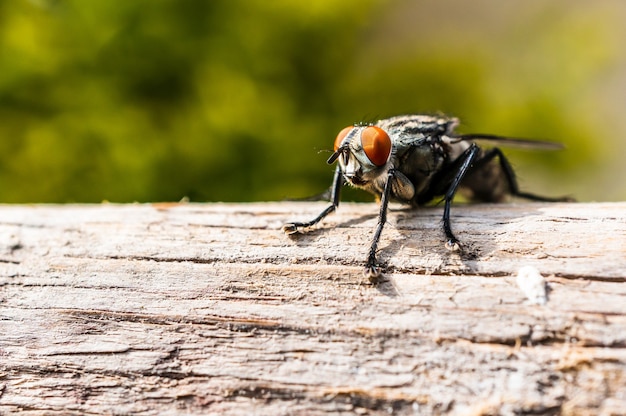A close-up photograph captures a fly perched on a light brown log with dark brown splotches and some bark visible. The fly, facing slightly to the left, has striking reddish-orange eyes that dominate its face, which features a mixture of beige and green. The rest of its body is primarily black and dark gray, with some white hairs on its legs. Three of its legs are clearly visible in the foreground, while another leg is barely seen at the back edge of the log. One of the fly's black-tipped wings is extended. In the blurry background, there's a soft focus of light and dark green leaves, hinting at distant trees with accents of yellow. The log is horizontally oriented across the image, providing a detailed, in-focus contrast to the out-of-focus backdrop.